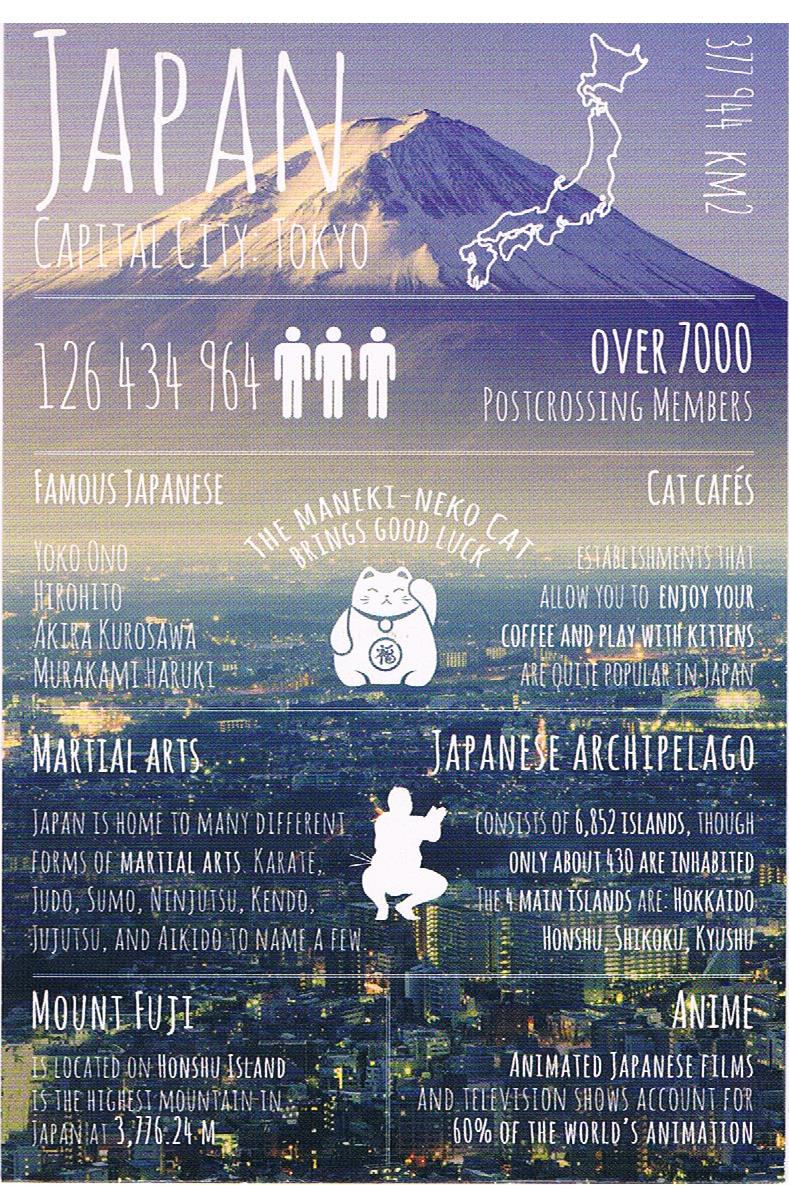This is a detailed brochure or poster depicting an aerial view of Japan, prominently displaying a densely packed city at the bottom and a snow-capped Mount Fuji at the top. Overlaid in white text are various intriguing facts about Japan: it highlights Tokyo as the capital city, includes an outline illustration of the country, and mentions its population and postal code 126-4349-964. The image features notable figures like Yoko Ono, Emperor Hirohito, Akira Kurosawa, and Haruki Murakami. At the center, there is an illustration of a Maneki-neko (good luck cat) and information about popular cat cafes. Additionally, the brochure details Japan's rich tradition in martial arts, listing forms like karate, judo, sumo, ninjutsu, and kendo. It emphasizes the Japanese archipelago, consisting of 6,852 islands with only about 430 inhabited, and the four main islands: Honshu, Hokkaido, Kyushu, and Shikoku. Mount Fuji, Japan's highest peak at 3,776.24 meters, is also featured. Lastly, it notes that anime, Japanese animated films, and TV shows make up 60% of the world's animation.